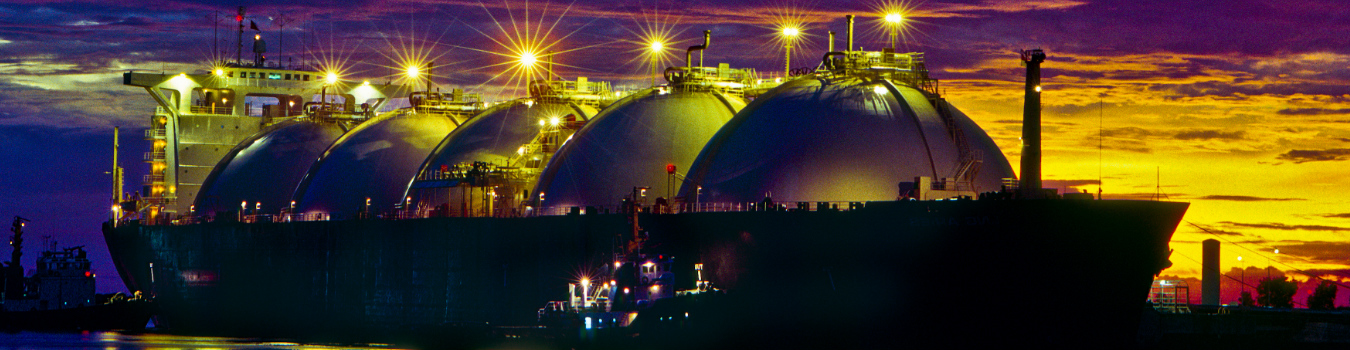This captivating dusk photograph showcases a massive tanker ship dominating the scene, spanning nearly the entire length of the frame. The ship's imposing presence is accentuated by its sleek black hull, contrasted by a white section at the stern, likely housing the captain's quarters. The sky is a dramatic blend of yellow and purple hues, with a sunlit right side transitioning into clouds painted in rich purples and oranges across the top and left of the image. The tanker features five formidable gray metal half-dome structures, each marked with lights and topped with walkways, possibly housing fuel cells. These domes are so large that each is comparable in size to the smaller ships flanking the tanker. One of these accompanying vessels is brightly illuminated, while the other remains shadowed, adding depth to the twilight maritime scene.